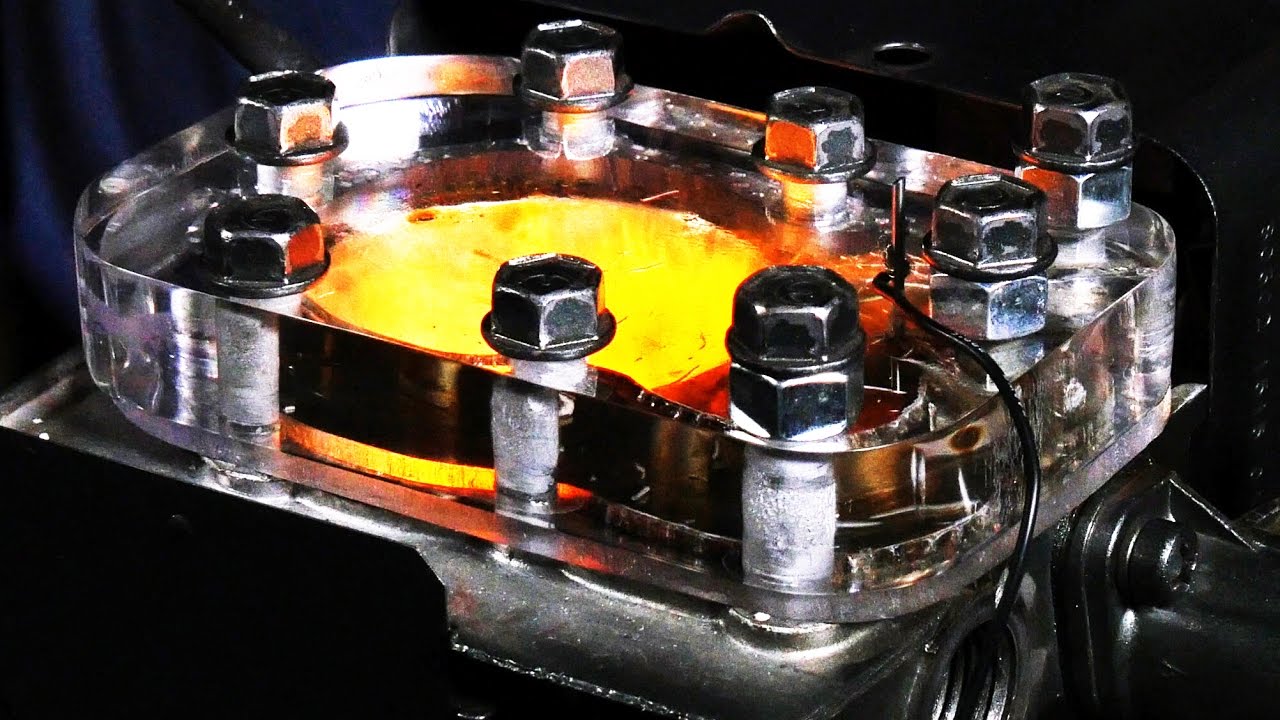The image depicts a detailed and seemingly complex device, primarily silver in color, possibly a smelter or an engine component. This device features a central section that glows red-hot and molten, emanating a yellowish-reddish fiery glow. Surrounding this central area are nine visible bolts and screws, which secure a large, clear plexiglass plate to the top of the device. The plexiglass allows visibility of the fiery inner workings. A black wire extends from a lower area, threading its way up to an attachment point between two bolts on the metal surface. The setup is framed by dark elements, enhancing the contrast of the chrome, yellow, orange, and black hues. Overall, the assembly appears both functional and artistic, suggesting it might be a practical device or a creative representation.